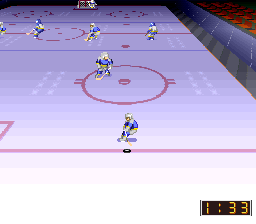This digital image captures a screenshot from a vintage hockey video game, characterized by pixelated graphics and gradient, less detailed lines. The scene displays a virtual hockey rink, which shifts in color from white at the forefront to light and then darker purple toward the background. Seven players, donned in blue, white, and yellow uniforms, are actively engaged in the game, skating across the ice and navigating around the red lines and circles typical of a hockey rink. In the upper right of the screenshot, a section of the background displays a mix of gray, blue, and red hues. Notably, in the lower right corner of the image, a standalone black digital timer reads "1:33".